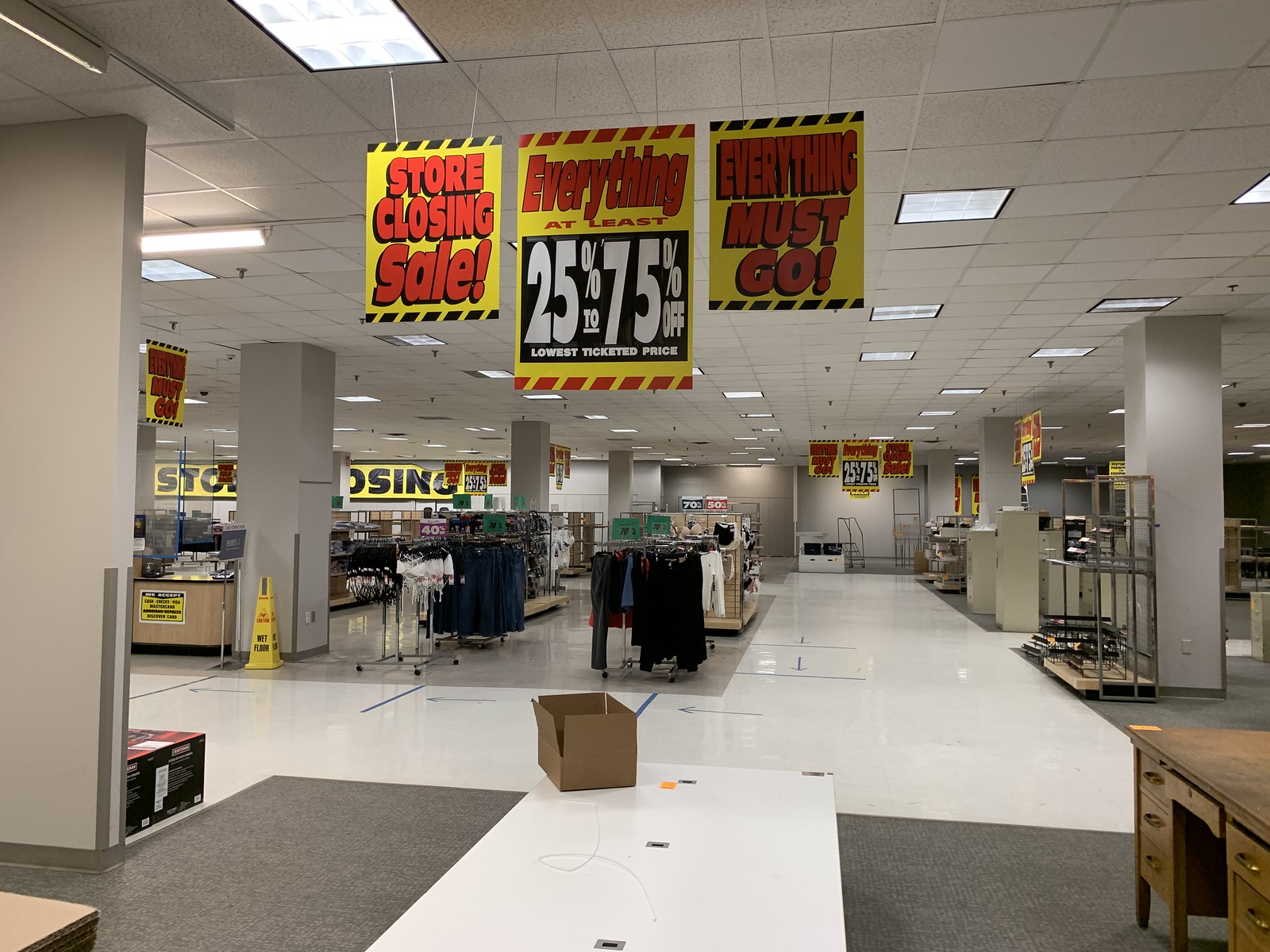The image depicts a spacious department store undergoing a "Store Closing" sale, characterized by bright yellow and red banners with black squares prominently displaying the message, "Store Closing Sale," announcing discounts of 25% to 75% off the lowest ticketed price, alongside the phrase "Everything Must Go." The store features a mix of white and grayish tiles on the floor, with a brown cardboard box conspicuously placed in the center. Above, the ceiling is composed of gray square panels. On the right side stands a wooden desk and gray column with shelving units, some of which are empty, suggesting the store's clearance efforts. The left side of the store houses filled clothing racks, including bikinis or underwear, emphasizing the varied merchandise being sold off. Despite the lingering items, the area feels notably vacant, indicative of its imminent closure.